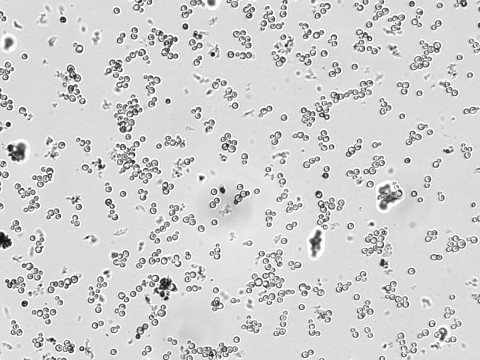The image appears to be a highly magnified black and white microscopic view, possibly of a micro-organism. The entire scene is composed of numerous small, irregularly shaped circles that closely resemble cells. These circles vary slightly in size and are scattered across a predominantly light gray background, with some areas appearing darker and more clustered towards the center. Within the clusters, some circles appear to glow, while others are outlined in black, adding contrast. The background also contains subtle smudges and blur, creating a textured effect. While most of the circles are sharply defined, several are out of focus, contributing to the overall intricate and detailed composition of the microscopic landscape.